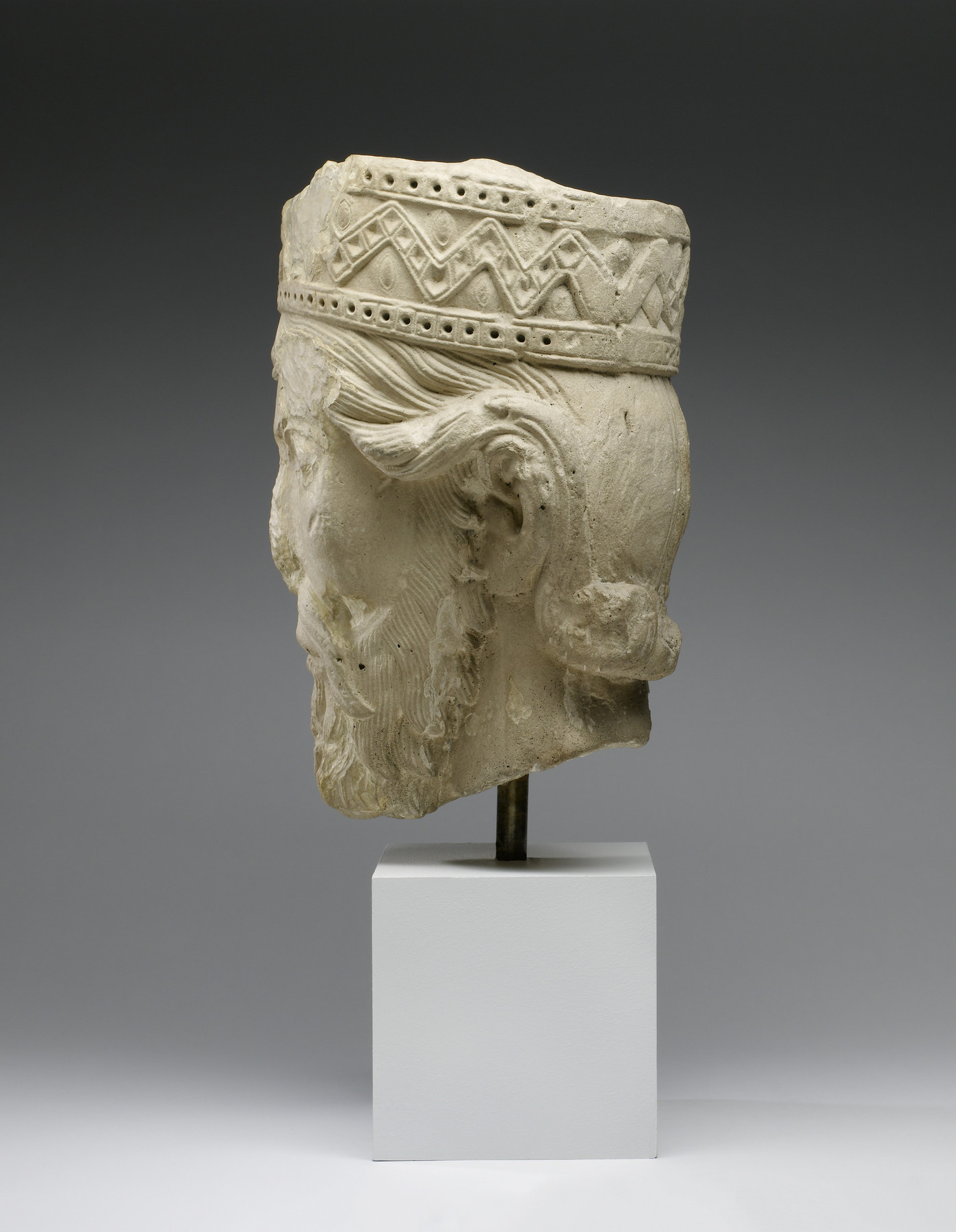The image depicts a stone bust of a man, likely an emperor, positioned on a slender metal rod that is fixed into a white cube base. The statue showcases a left-profile view of the man, whose face is marked by a notably eroded nose. He dons a flat, cylindrical crown adorned with vertical and horizontal zigzag patterns intermixed with dots. The man's wavy hair flows back and curls upwards just above the nape of his neck, partly covering his ear. A full beard extends down to his chin line. The bust, which appears to be sculpted from a lightly colored, aged stone, is set against a dark gray background, suggesting a museum display.